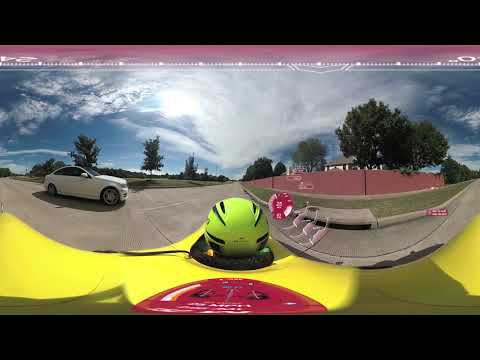The screenshot, taken from a race car driving video game, presents a panoramic view from the perspective of a yellow race car being driven by a person wearing a green helmet with black stripes. The helmet is prominently visible, just peeking above the car's top. The car, adorned with a partially visible red or yellow logo, speeds down a two-lane street on a bright, clear day with a blue sky dotted by large white clouds. To the left, a white BMW sedan passes by, while both sides of the road are lined with lush grass and large trees. A distinct red fence runs along the right-hand side, behind which stands a white building with a gray roof. There's also a sidewalk and a brick wall on either side in parts of the scene. Click marks indicating distance can be seen at the top of the screen, and next to the helmet, a round dial functions as a speedometer. The road appears slightly distorted in the image, with a swooping effect that draws the eye along the racing path.